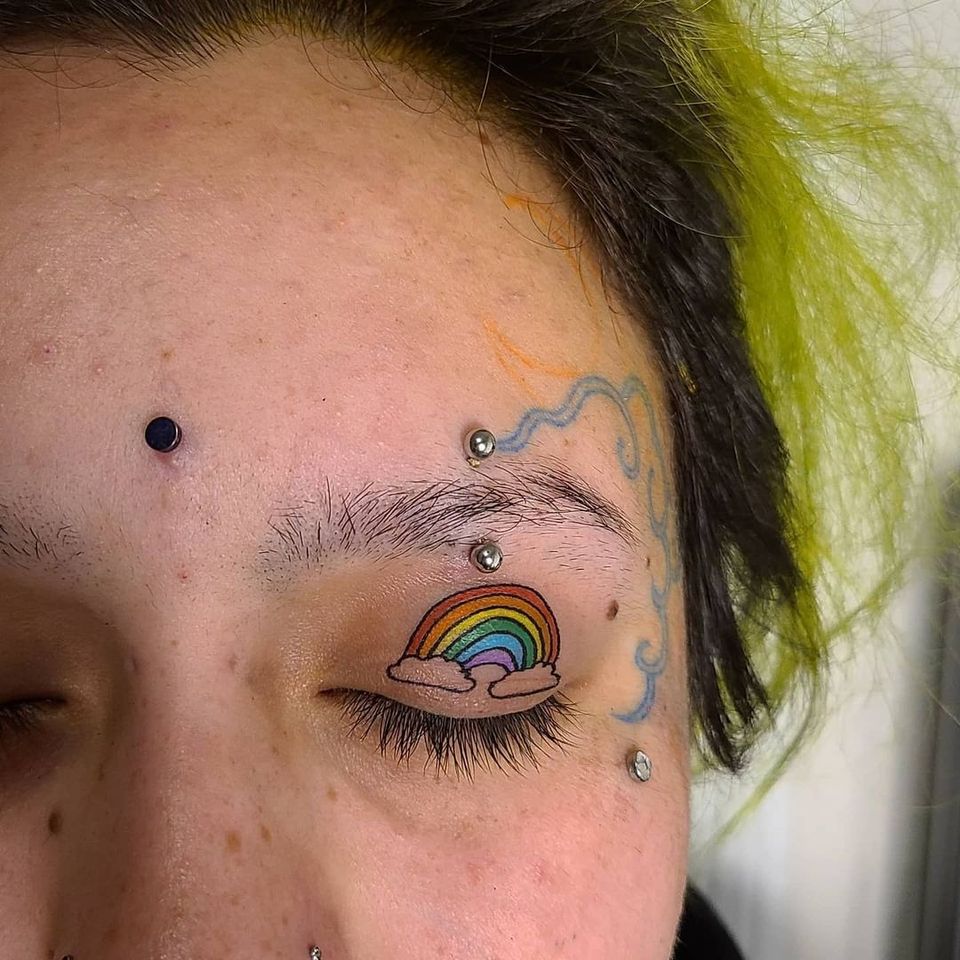The image features an extreme close-up of a woman's face, capturing the area from the top of her head down to the bridge of her nose. Her hair is primarily dark brown with sections dyed a vivid green. Visible in the image are multiple facial piercings: a small black metal stud between her eyebrows, a silver ball just below her left eye, and another piece of metal jewelry piercing her sparsely haired eyebrow. Radiating from the silver ball piercing is a blue squiggly tattoo that extends down around her temple to the side of her eye. Additionally, an orange squiggly tattoo can be seen intertwined with the blue one. Her left eyelid is closed, adorned with a colorful rainbow tattoo. The close proximity of the photo highlights the fine details of her skin, including visible pores.